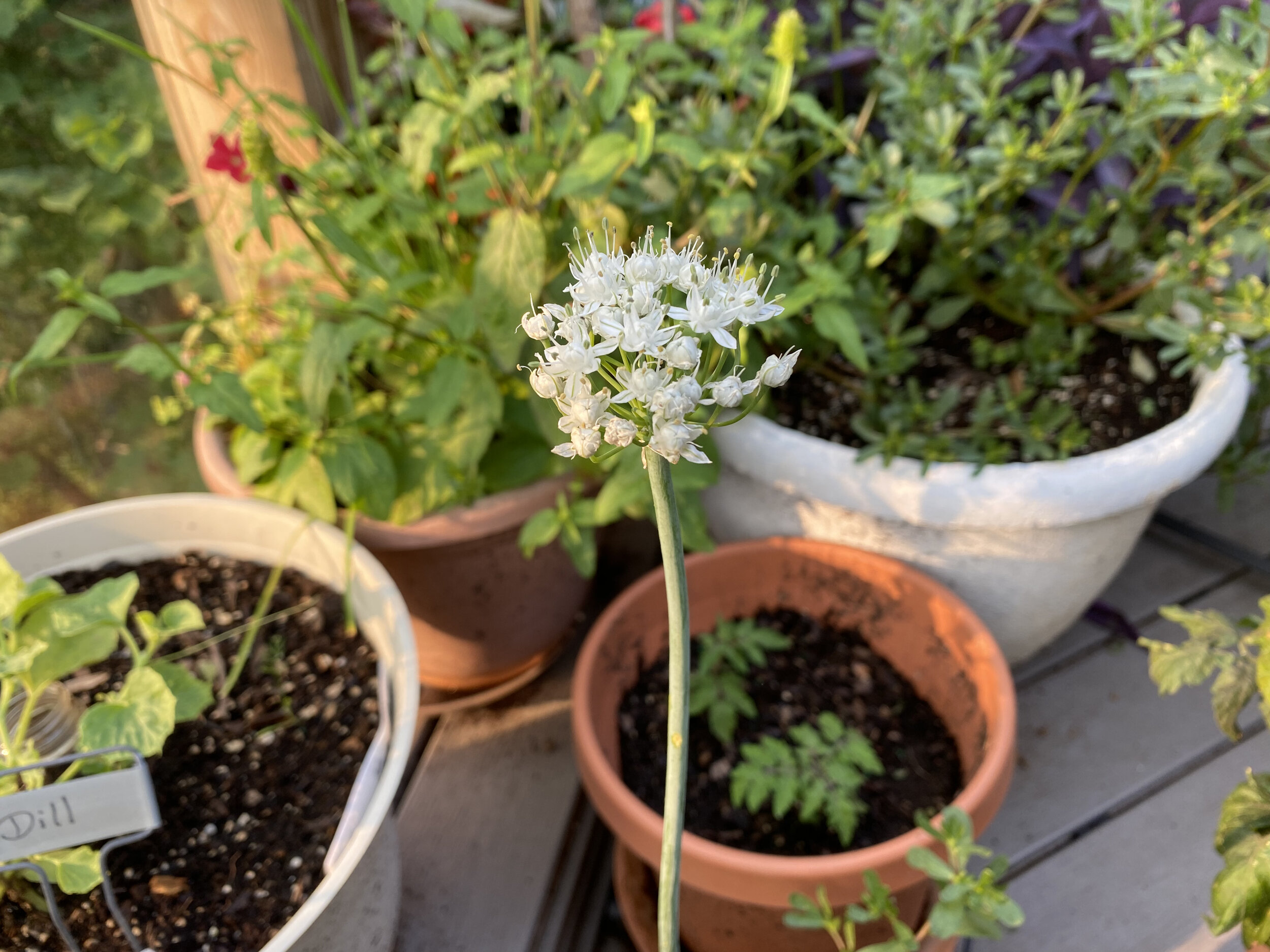This outdoor photograph captures a detailed arrangement of potted plants displayed on a gray wooden deck. Starting from the bottom left corner, there's a whitish pot with a small immature plant, labeled with a sign that reads "dill". Directly to its right, near the bottom center, is a smaller clay pot containing some blackish-brown dirt and a few green leaves. Just above this clay pot, slightly to the right, there is another clay pot, fuller with foliage, including a small red flower that adds a pop of color to the scene. In the upper right corner, one can see a larger, round, white pot brimming with unidentified greenery. Dominating the central part of the image is a tall, grayish-green stalk that emerges from the bottom, crowned with a cluster of delicate white flowers, highlighting the inherent beauty of gardening. The serene setting of this outdoor space showcases someone’s dedication to cultivating a variety of plants.